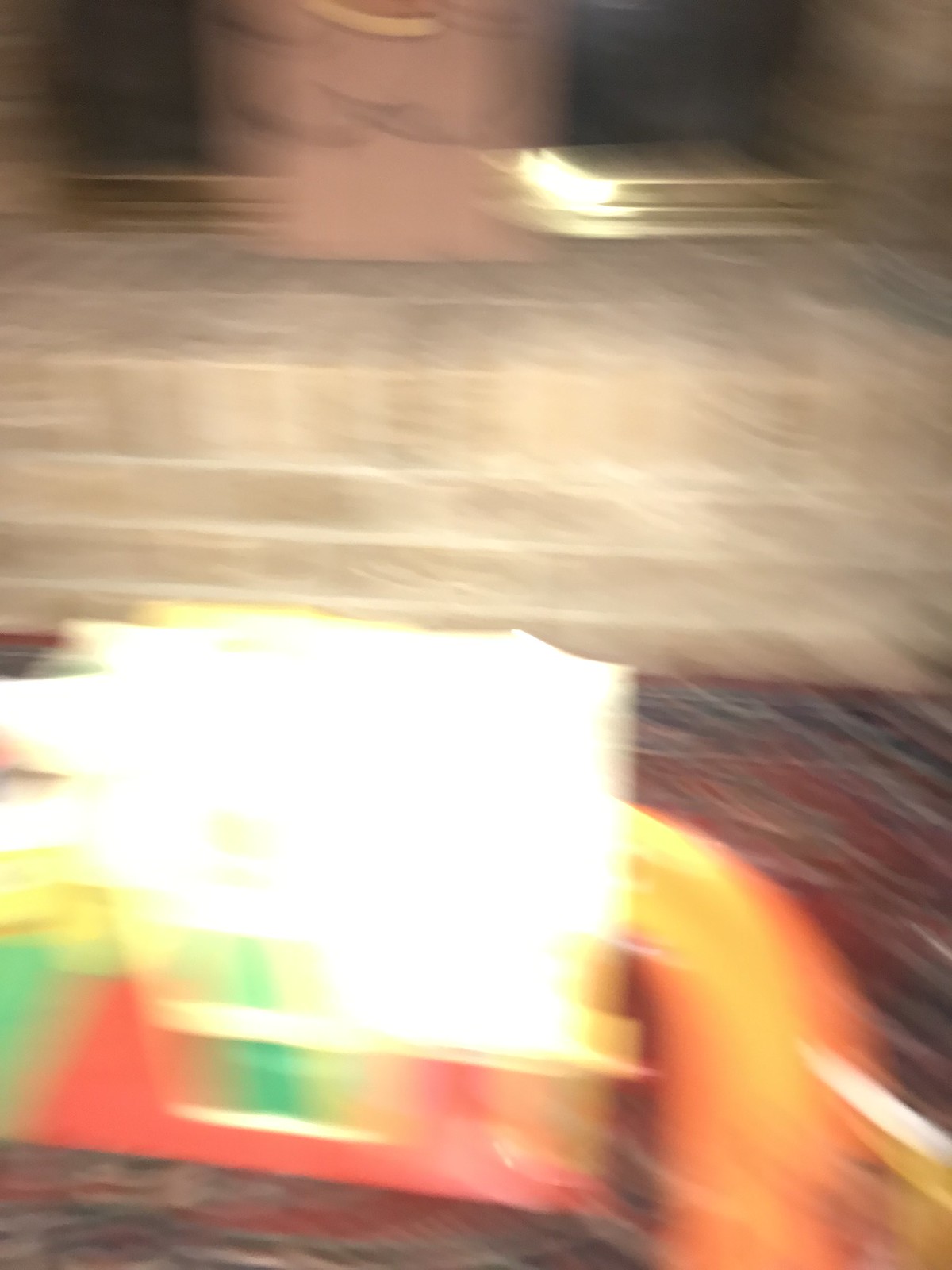The image is quite blurry, making it challenging to discern specific details. In the foreground, an object sits close to the camera with a red and green base. The top of this object is difficult to make out due to bright, reflective light obscuring its details. To the right of this object, there is an orange smear whose identity is unclear. The scene appears to be set on a carpet adorned with red and black patterns. In the background, a set of stone stairs with approximately four steps is visible. On the top step rests a pinkish box, while atop the stairs, there are golden, platform-like objects, one of which is shining. A black area is visible behind these golden platforms.